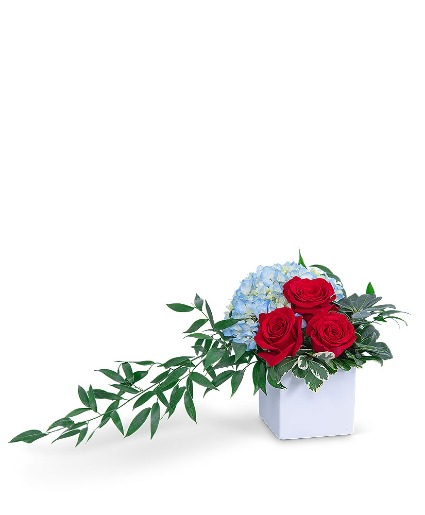This is a detailed photograph with an all-white background, featuring a square, white ceramic vase positioned slightly diagonally, allowing a view of both its front and side. The vase holds three vibrant red roses arranged in a triangular formation. Behind these roses, a large cluster of delicate, bluish-white flowers adds depth to the composition. The arrangement includes long, green stems and vine-like branches adorned with thin, oval, pointy green leaves, particularly jutting out prominently to the left side and casting a shadow on the surface. The entire display appears freshly watered and meticulously arranged, with the green leaves and vivid flowers contributing to a healthy and lively presentation.